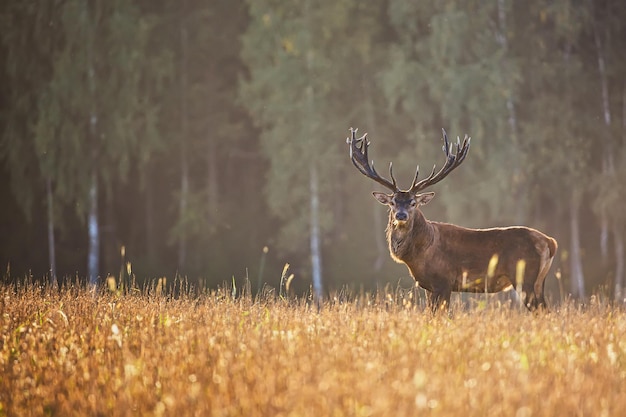This is a detailed color landscape photograph capturing a majestic male elk standing in an open pasture of tall, overgrown grasses that display hues of golden, tan, brown, and a hint of green. The elk, with its body facing the left and its head turned towards the viewer, gazes directly at the camera. Its impressive rack of antlers, featuring four central tines between the two main branches, extends gracefully to both sides of its head. The elk's coat is a blend of cream, brown, black, and tan shades, with lighter tones around the shoulder area and back end. It is chewing on a piece of grass and has prominent, outward-facing ears. In the background, a dense, out-of-focus forest of tall green trees, some with white trunks that are likely birch, provides a natural frame for this scene. The setting appears to be early fall, as the grass shows signs of starting to die, yet the trees remain fully leafed. This moment is frozen in daylight, capturing the tranquil and realistic beauty of wildlife in its natural habitat.